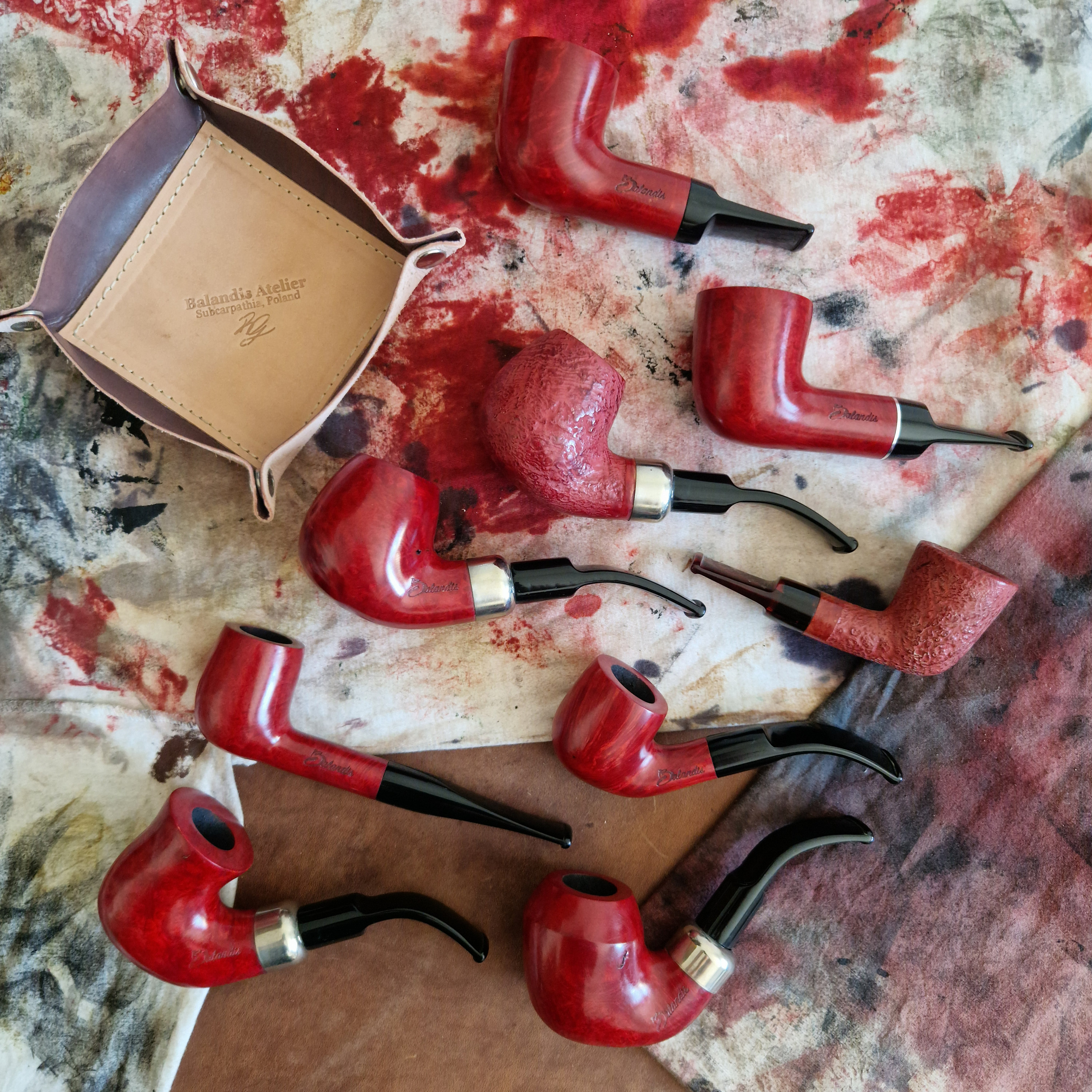The photograph depicts ten smoking pipes, reminiscent of those associated with Sherlock Holmes, positioned on a white cloth heavily stained with smeared and dropped paint in shades of red, gray, and black. The pipes vary in shape, with some featuring bent stems and others straight shafts. Their bowls range in size, with some being larger and others more petite. Most of the pipes have a glossy, brownish-red finish, though two exhibit a notably rough texture. Additionally, their designs include silver rings around the bowls and black mouthpieces. A brown leather pouch with a square bottom and pinched corners, bearing some illegible writing, rests in the upper left corner, suggesting it might be intended for storing the pipes, although it appears too small to hold all of them. The scene gives the impression of a workspace where pipes could be made or restored, as suggested by the colorful paint smudges on the cloth. In the upper right corner, there's a white box potentially indicating the pipes' brand, though its label is unreadable.